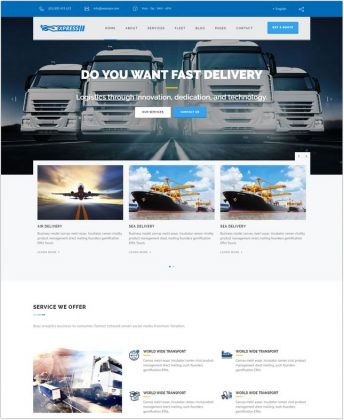In the banner of this logistics company's website, a crisp blue bar tops the page, featuring blurred white details that appear to include contact information and sharing options. Below it, a white tab featuring the company's logo, partially discernible with the word "Express," stretches across the header but doesn’t span the full width of the page. The navigation links on this tab are also blurred.

Dominating the banner, a vivid image showcases four sleek, white trucks with dark windows, all driving forward on a clear road with their lights on, symbolizing the company's promise of fast and efficient delivery. Superimposed on this image is the tagline, "Do you want fast delivery?" followed by "Logistics through innovators, dedication and technology" in white text, highlighting the company's commitment to cutting-edge solutions.

Further down, the page features three additional images: one of an airplane taking off, and two of the same industrial ship equipped with yellow cranes, each linked to presumably relevant content or posts. Below these images, there's a section titled "Services We Offer," although the specific services listed are too blurry to read.

At the page's bottom, a smaller, less distinct image of another truck is accompanied by selectable options, though, like the rest, it remains too blurry to discern specific details.